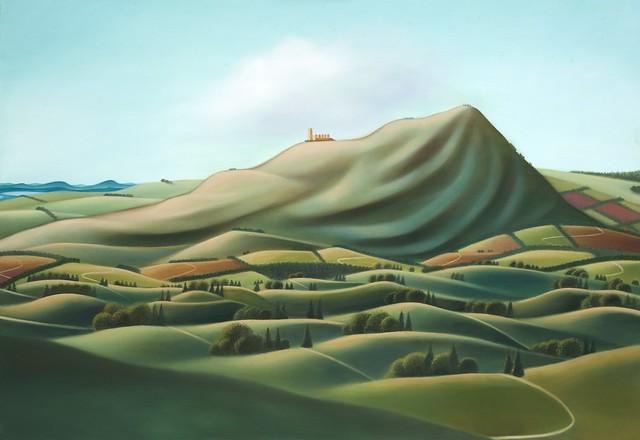The image is a detailed digital illustration of a serene countryside landscape depicted as a piece of cartoon artwork. Dominating the scene is a large hill or mountain, centrally located, colored in shades of green and brown. Atop this hill sits a factory-like structure with five smokestacks and an additional tall, indiscernible structure. The foreground features smaller, rolling green hills interspersed with patches of brown and red farmland. There are clusters of trees, including tall, triangular pine trees and full, rounded trees with scattered leaves. On the left side, there is a body of water colored blue, while on the right side, a row of trees lines the background. The sky is a clear light blue with minimal clouds, including one prominent cloud in the center. The scene is devoid of vehicles, animals, or people, highlighting the natural, unspoiled beauty of the landscape. The colors used predominantly are various shades of green, brown, light blue, and touches of red.